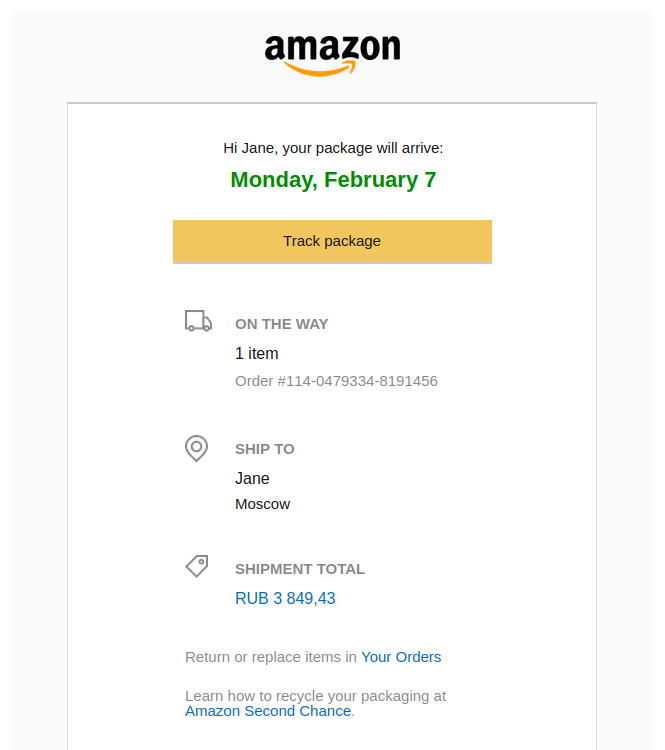**Detailed Caption:**

This screenshot captures an email notification depicting a delivery update from Amazon. The email is enclosed within a light gray border at the very top. Positioned at the top center of this email, the word "Amazon" is prominently displayed in black font. Below the text, the iconic Amazon logo, featuring a yellow arrow curving to the right, is distinctly visible.

Directly beneath the logo, against a white background, the email addresses the recipient with the greeting "Hi Jane" followed by a delivery notification in bold black font: "Your package will arrive." Highlighted in red font, the specific delivery date is stated as "Monday, February 7th."

Following this, an actionable orange rectangular button with the text "Track Package" written in black font invites the recipient to monitor the delivery status.

Underneath the button, a gray icon of a truck is presented with the accompanying gray text "On the way." Below this section, the text "1 item" appears in bold black font, indicating the number of items being shipped. Additionally, the order number "Order #114-0479334-8191456" is provided in gray font for reference.

Further down, a gray location icon signifies the shipping address, labeled "Ship to" in gray font. Directly below this, the text "Jane, Moscow" is displayed in black font indicating the recipient's name and city of delivery.